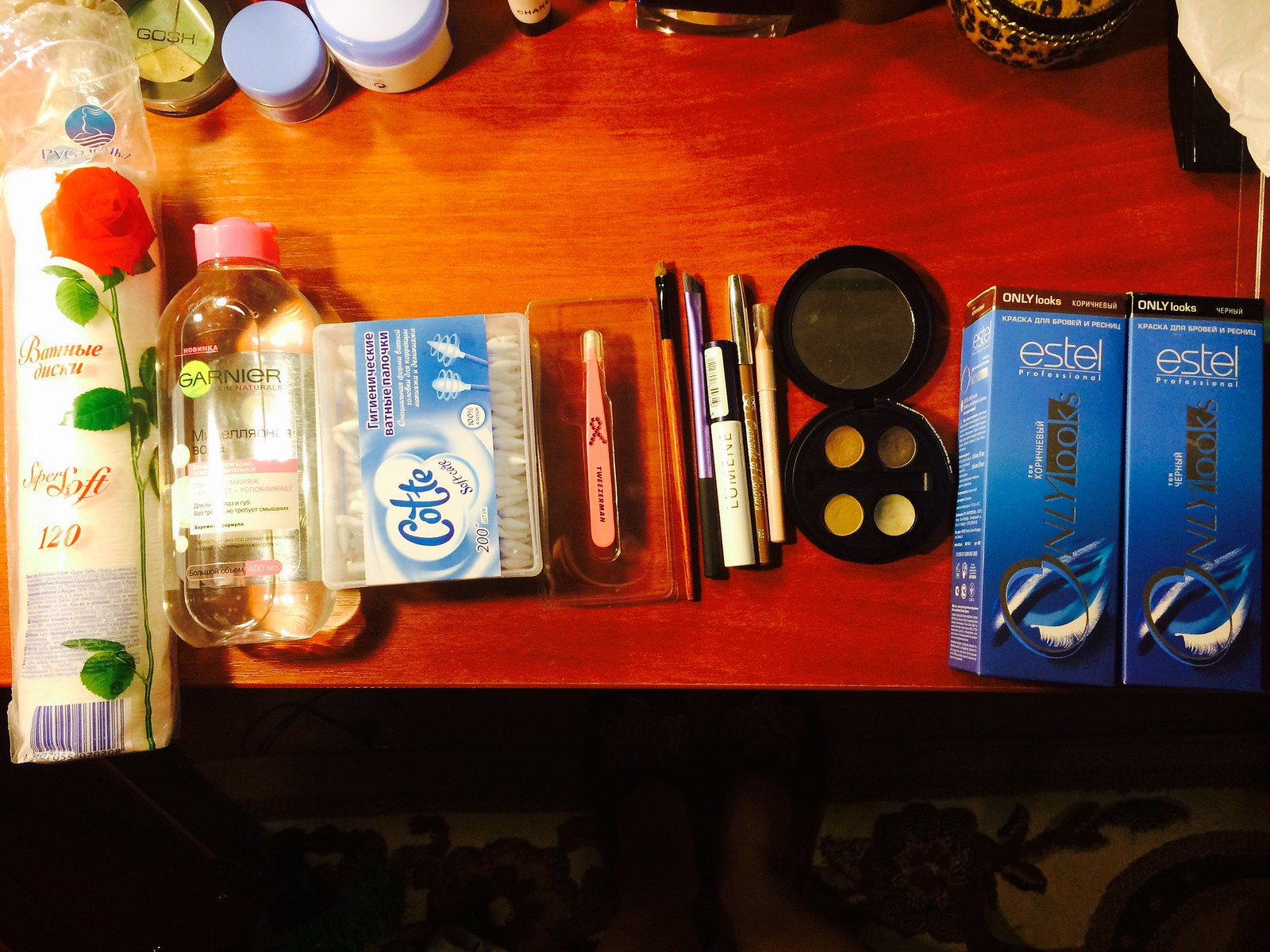On this dark reddish stained table lies an array of skincare and makeup products, each neatly arranged. Starting from the left, there is a round plastic container filled with circular makeup remover pads. Next to it stands a clear plastic bottle with a pink lid, labeled "Garnier," possibly containing makeup remover liquid. Adjacent to that is a package of Cottee cotton balls, featuring both round and pointed cotton balls depicted on the packaging. To the right, a pink makeup brush with a white tip, ideal for applying eyeshadow, rests alongside a few additional brushes and possibly a concealer. Toward the far right of the table, two unopened blue boxes bearing the name "Estelle" in white letters lie side by side. The collection provides a comprehensive assortment of tools for facial care and makeup application.